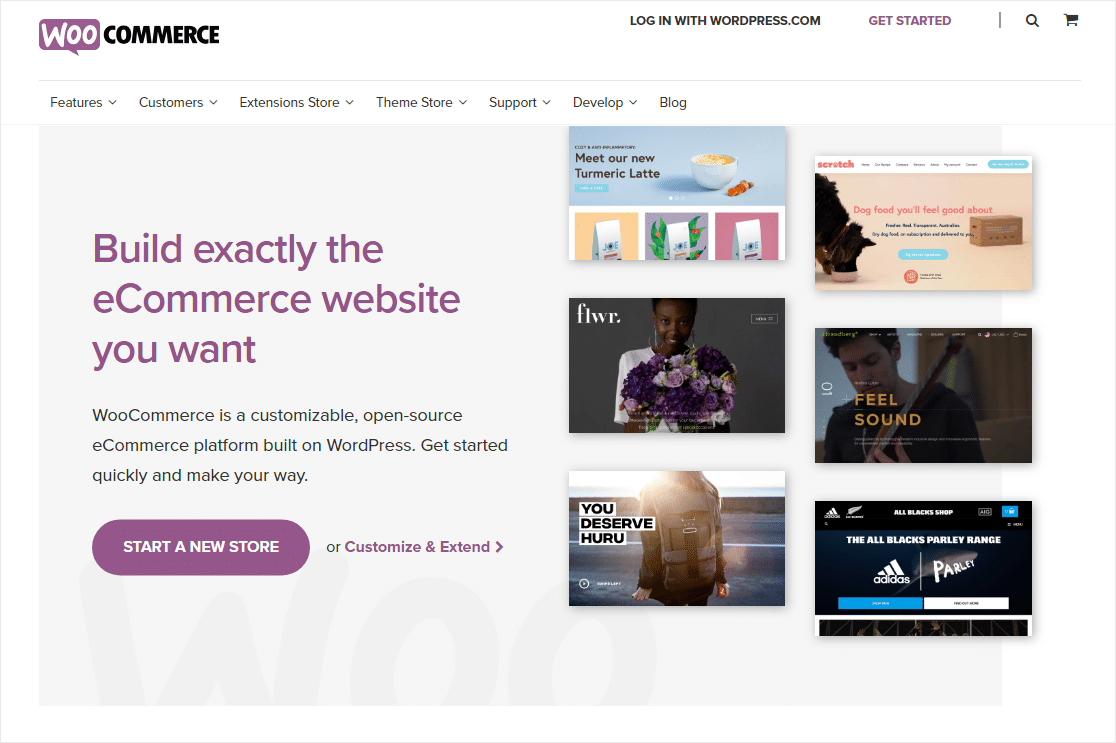The image showcases a screenshot of the WooCommerce homepage on a white background. At the top, “WooCommerce” is prominently displayed, with “Woo” written in white font on a purple rectangle, and “Commerce” in black font.

The page features a login option labeled “Login with WordPress.com” and a prominent call-to-action button reading “Get Started,” which is highlighted in purple. There are icons for a magnifying glass and a shopping cart, indicating search and shopping functionalities respectively.

Navigation options are clearly listed, including "Features," "Customers," "Extensions," "Store," "Theme Store," "Support," "Develop Blog," and a tagline that reads, "Build exactly the e-commerce website you want." WooCommerce is described as a customizable, open-source e-commerce platform built on WordPress. 

Further down, there's a large purple oval button that says “Start a New Store” in white text. This is followed by text blocks and six rectangular images promoting various products:
1. "Meet Our New Turmeric Latte"
2. "FLWR"
3. "You Deserve Huru"
4. "Dog Food You’ll Feel Good About"
5. "Feel Sound"
6. "The All Blacks Parley Range by Adidas and Parley"

The site highlights WooCommerce's flexibility in allowing users to customize, extend, and build their e-commerce platform to meet specific needs.